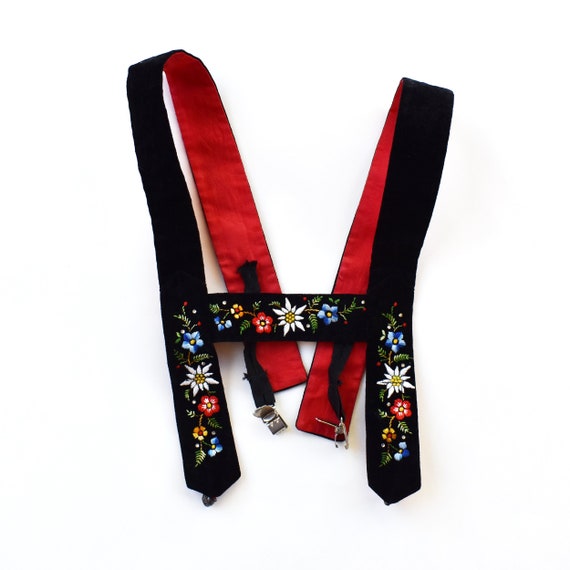This image showcases a set of traditional German suspenders, typically paired with lederhosen. The suspenders are predominantly black with a silky red lining on the inside, a feature that visually suggests a similarly silky texture on the outside. They are intricately detailed with vibrant floral embroidery, displaying a variety of colorful wildflowers—including shades of blue, white, red, yellow, and green foliage—on both the vertical and horizontal straps. The silver clasps at the bottom of these black straps are notably shiny and are designed for attaching the suspenders to pants. The H-shaped configuration of the suspenders includes a horizontal strap that unites the two vertical straps, each adorned with embroidered flowers. This detailed piece is set against a pure white background, enhancing the vivid colors and intricate details of the embroidered flora.